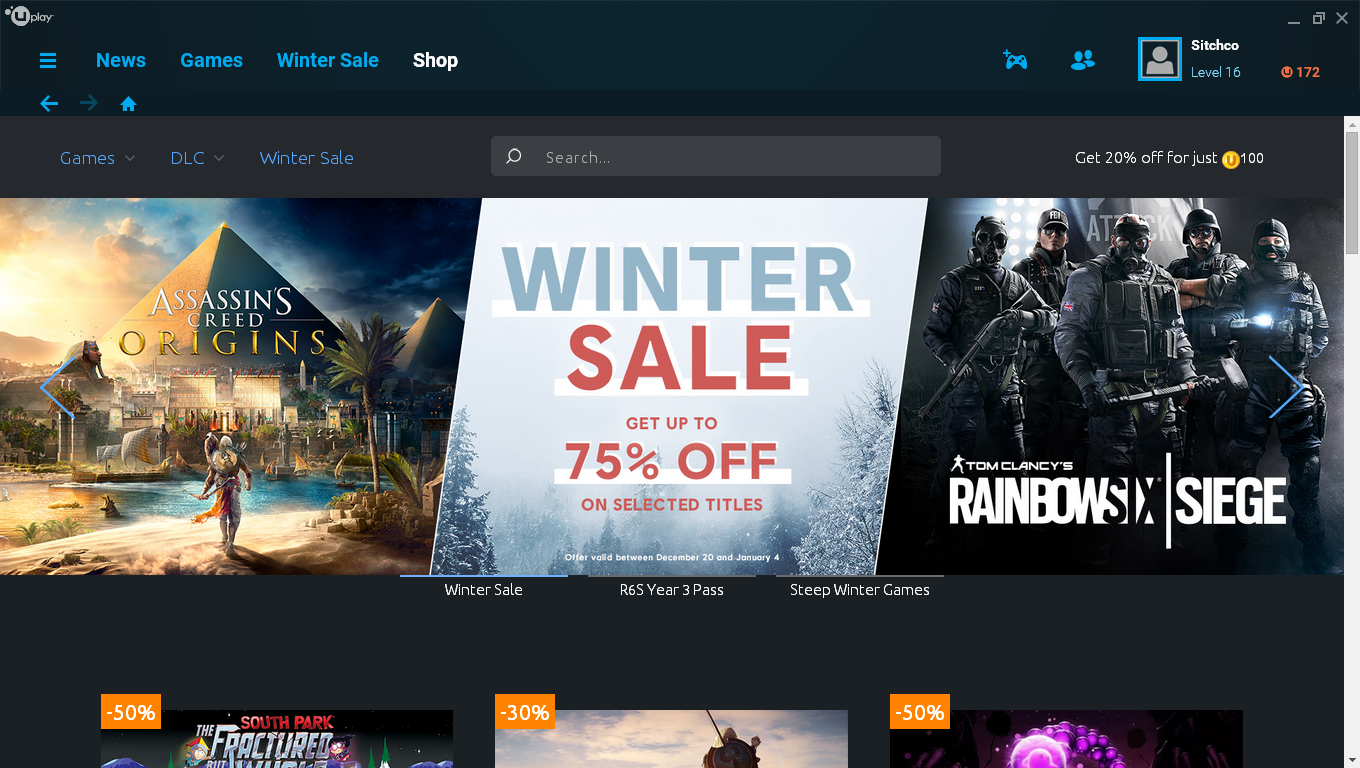A detailed, cleaned-up caption for the image:

"A screenshot from the Uplay website, showcasing a vibrant advertisement for their winter sale. The sale banner prominently announces discounts of up to 75% on selected titles, displayed against a dark mode background with black and very dark gray hues. The screen is populated with various game advertisements arranged somewhat haphazardly, with some images cut off due to the zoomed-in view. In the top-left corner, the Uplay logo stands out in gray, accompanied below by a navigation bar offering options such as News, Games, Winter Sale, and Shop. On the right side of the screen, the standard window control icons for minimizing, maximizing, and closing the window are visible, along with additional icons including the user profile. The profile section reveals that the user, named Sitchko, is currently level 16 with 172 points. Also visible is a sub-banner featuring links to Games, Downloadable Content, and the Winter Sale, providing further navigation options."